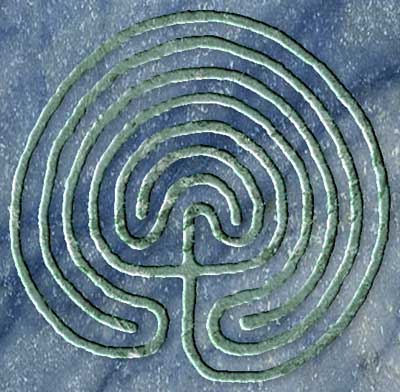The image depicts an intricate, abstract design resembling a labyrinth, set against a blue, marble-like background with white speckles and darker blue channels. The maze-like pattern, rendered in shades of green and teal with some white outlines, features a rounded shape with a cross at its center, suggesting no true entrance or exit. The lines of the design spiral outward from the middle, creating gaps and curves that give it a complex, looping appearance. The bottom part of the pattern includes an upward-curving line, adding to the sense of depth and movement. Despite its maze-like appearance, the structure ultimately leads to a dead-end in the center, hinting more at a symbolic or emblematic purpose rather than a functional maze.